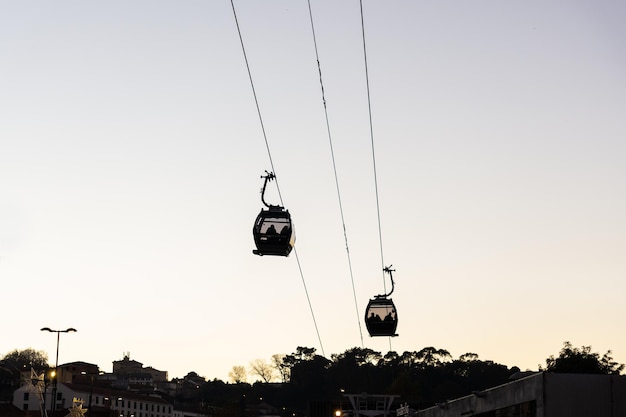In the photograph, two gondola-style cable cars ride on separate cables, with an empty cable between them. The left gondola is positioned higher, while the right gondola is lower, creating a slight diagonal tilt where the cables extend from the bottom center of the image up towards the top center, slanting left to right. Silhouettes of people can be discerned inside each gondola – two in the left and three in the right. These glass-enclosed cars are connected to the cables by L-shaped arms, with the left arm reaching from the gondola's top and the right arm from its bottom. The scene appears to be captured just after sunset, characterized by a striking sky that transitions from a soft yellowish-orange at the horizon to a darker blue above. In the lower portion of the image, you can observe the silhouettes of a bridge, streetlights, a white fence, and three buildings, all set against the evening sky. The silhouetted tree line at the bottom completes the picturesque view of what looks like a serene city or small town.